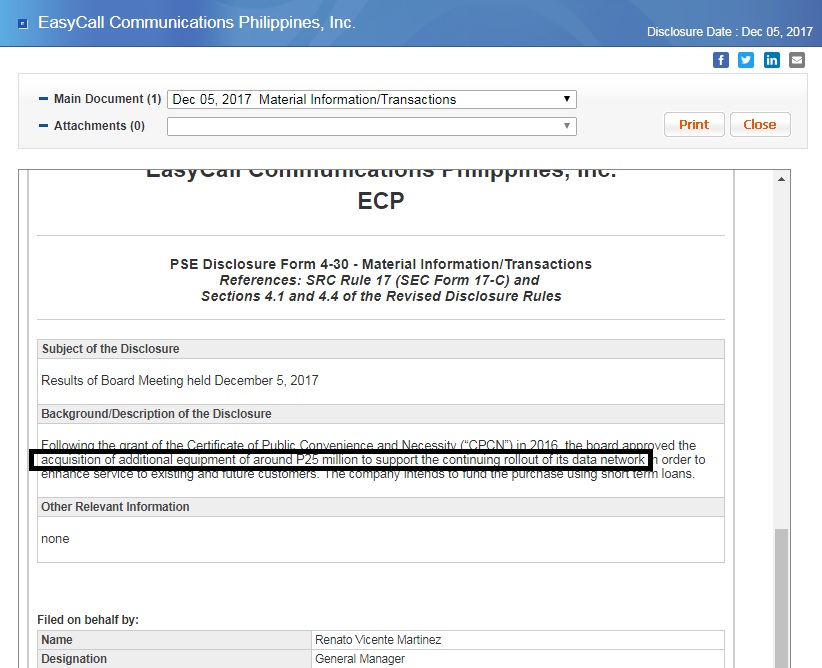This image depicts a webpage belonging to EasyCall Communications, Philippines, Inc. The page prominently displays the company's name, with the disclosure date noted as December 5, 2017. The top section of the website is adorned in gray, providing a sleek background for the content.

On the right-hand side, there are social media icons including Facebook, Twitter, LinkedIn, and an envelope icon set within a brown square, signaling the presence of contact or share features. The main document on the page is titled "Material Information/Transactions," dated December 5, 2017. However, the attachments bar beneath this title is empty.

The right tab of the page features print and close buttons, allowing users to either print the document or close the webpage. The website text is styled in orange, including the company's name, which is depicted as "EasyCan Communications, Philippines, Inc." but clarified to be "EasyCall Communications, Philippines, Inc." hyphenated as ECP, where the letters appear cut off at the top of the page.

A PSE disclosure form is included, describing the nature of the disclosure. The subject of the disclosure is listed as the results of a board meeting held on December 5, 2017. In the background description, it details that following the grant of a certificate, the board approved certain actions outlined in a black box. The section labeled "Other Relevant Information" remains empty, with the text "none" indicating no additional details are provided. The form is filed on behalf of an individual whose name and designation are included towards the end of the document.